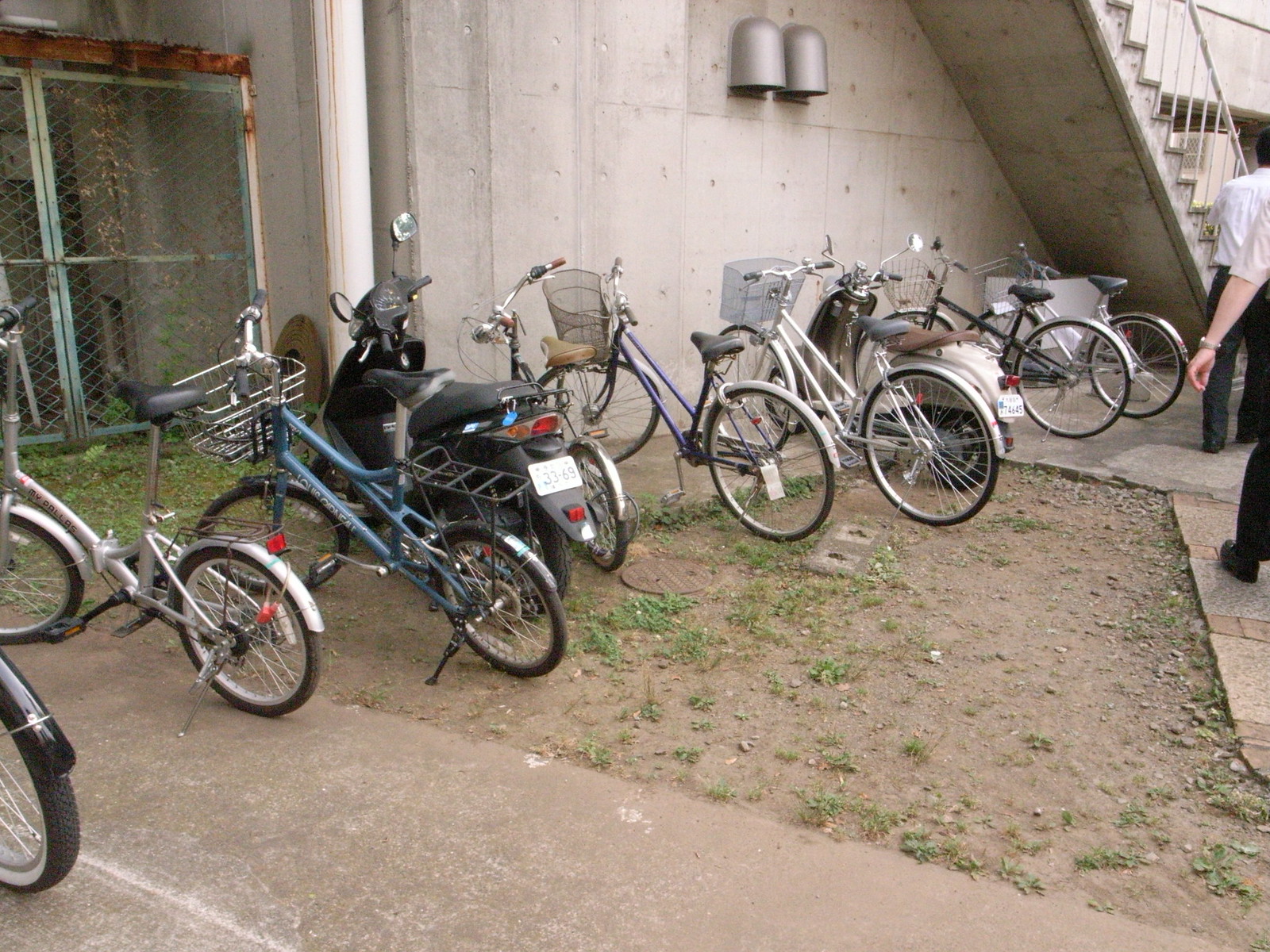This outdoor photograph features a concrete building with a fenced-in area and a white staircase ascending the side of the structure. Underneath the staircase, there are two cylindrical light fixtures attached to the wall, which is light gray. The building is bordered by a combination of pavement and asphalt walkways. In between the walkways, there's a sparse area of dirt and patchy grass, measuring around 10 feet by 10 feet, triangular in shape, with some short weeds scattered throughout.

The center of the image showcases a line of parked bicycles and motorcycles, mostly in silver, blue, and white colors. There are seven or eight bicycles, each equipped with metal baskets on the front and some with holders on the back. Among the bicycles, there is a black motorcycle with a red taillight and a white license plate bearing the number 3365. Additionally, there is another motorcycle, possibly white, mentioned in some accounts. 

On the far left, there's a rusted chain-link gate, and on the far right, two people are walking down the sidewalk. Both individuals are dressed in white shirts, black dress pants, and black shoes. One person has a silver watch on his left wrist. The entire scene is illuminated by daylight, capturing the realistic details of this utilitarian outdoor space designed for parking bicycles and providing pedestrian access.